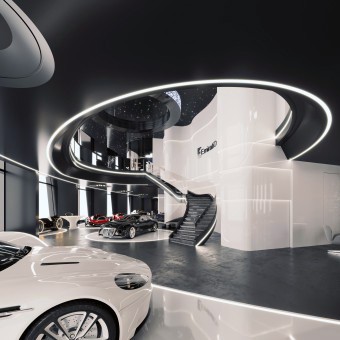The photograph captures the interior of a modern, high-end car dealership with a sleek, black and white aesthetic. The focal point of the image is a prominent black staircase in the center, leading up to a circular open space on the second floor, surrounded by white walls and LED lights. The ceiling above the staircase is predominantly black with white detailing. The ground floor is a combination of black and white tiled areas, with several prestigious sedans displayed. On the front left, there's a white car, possibly a Porsche, facing right. Near the black stairs to the left, there's a black car, potentially a Bentley or Cadillac. In the distance, another red car is visible, and closer to the staircase on the left side, there's yet another black car. The second floor features a black railing, and above, there appears to be a third floor with another half-circle design. The overall environment is futuristic, hinting at sophistication and luxury.